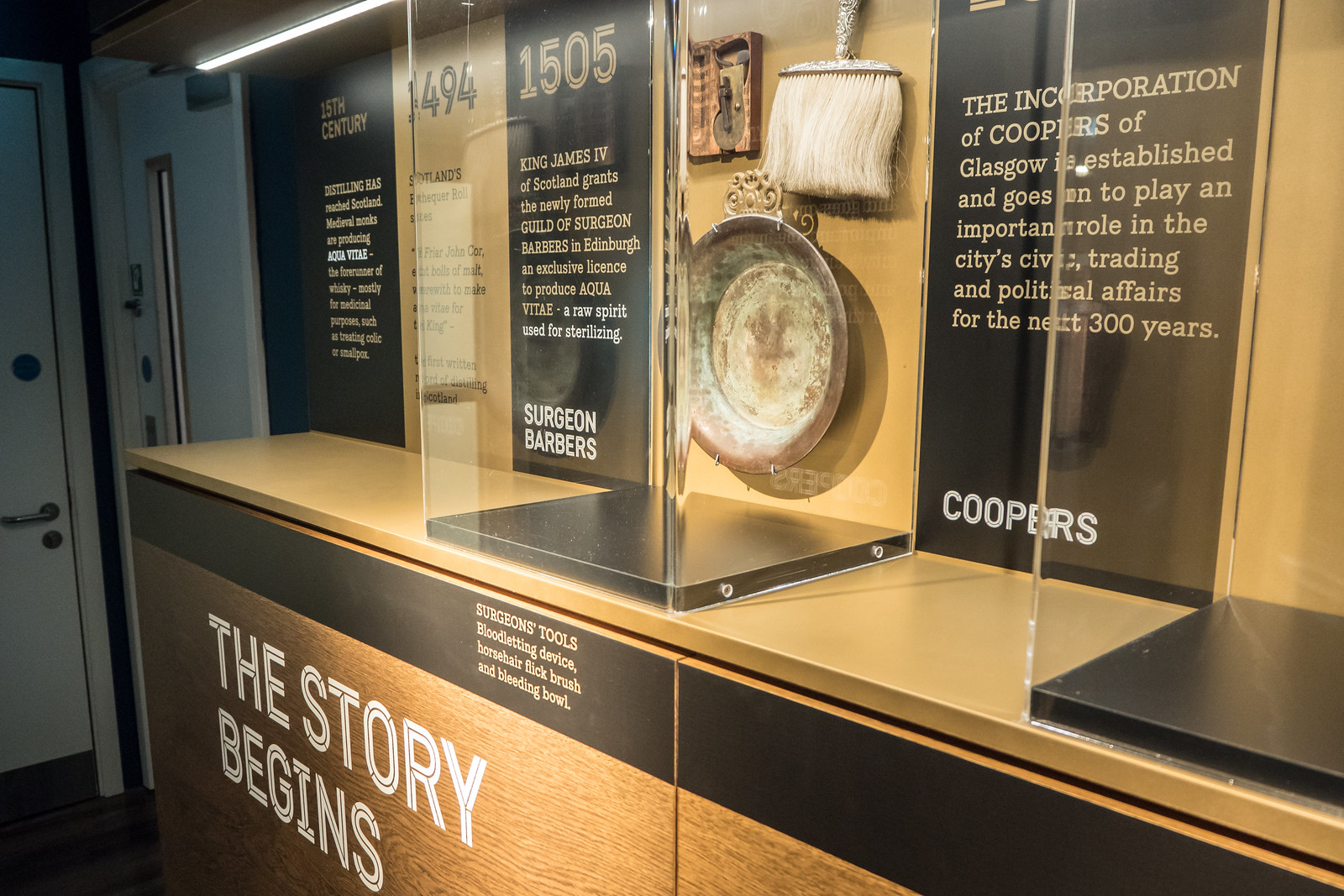The photograph captures a detailed display inside a museum, likely a Scottish museum dedicated to the history of barbers and Coopers (workers who make and repair wooden barrels). The focal point is a long display cabinet with glass front and built-in lighting. Front and center are historical tools, including a pan and a brush or broom. Prominently featured text within the display reads "The story begins," and elaborates on the historical significance of the Surgeons and Barbers, dating back to 1505, and the incorporation of the Coopers of Glasgow. This incorporation went on to play an important role in the city's civic, trading, and political affairs for the next 300 years. The photograph captures the detailed wood paneling of the cabinet, accentuating the historical importance of these artifacts. An exit door is visible to the left side of the image, adding context to the setting.